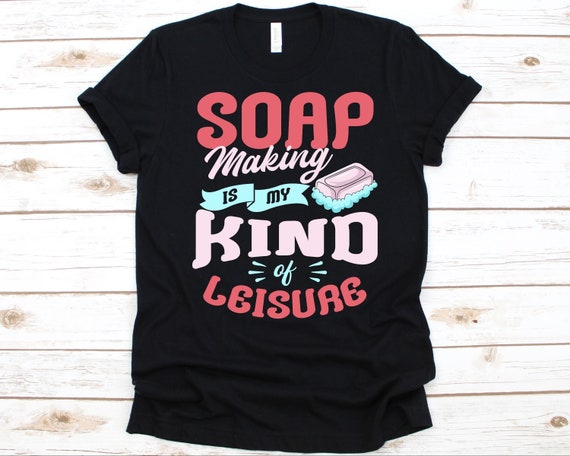In the image, a black graphic t-shirt is displayed on a weathered, light brown, almost beige wooden surface with horizontal, whitewashed planks featuring brown knots and edges. The t-shirt features a vibrant design where the text "Soap Making is My Kind of Leisure" is prominently displayed in a mixture of bright colors. The largest word, "Soap," is in a bright pink, while "Kind" is in a pale pink and also relatively large. The word "Leisure" is in the same bright pink as "Soap," and "Making" appears in a pale pink, script font within a square. The phrase "is my" is in black, all-caps font on a turquoise banner, while the word "of" is rendered in turquoise script, surrounded by six action lines. Additionally, there's an illustration of a soap bar with bubbles underneath it positioned to the right of the text. The short-sleeved shirt has its sleeves rolled up and a white rectangular tag is visible inside the neck. The shirt is not laying completely flat, giving it a casual, relaxed appearance.